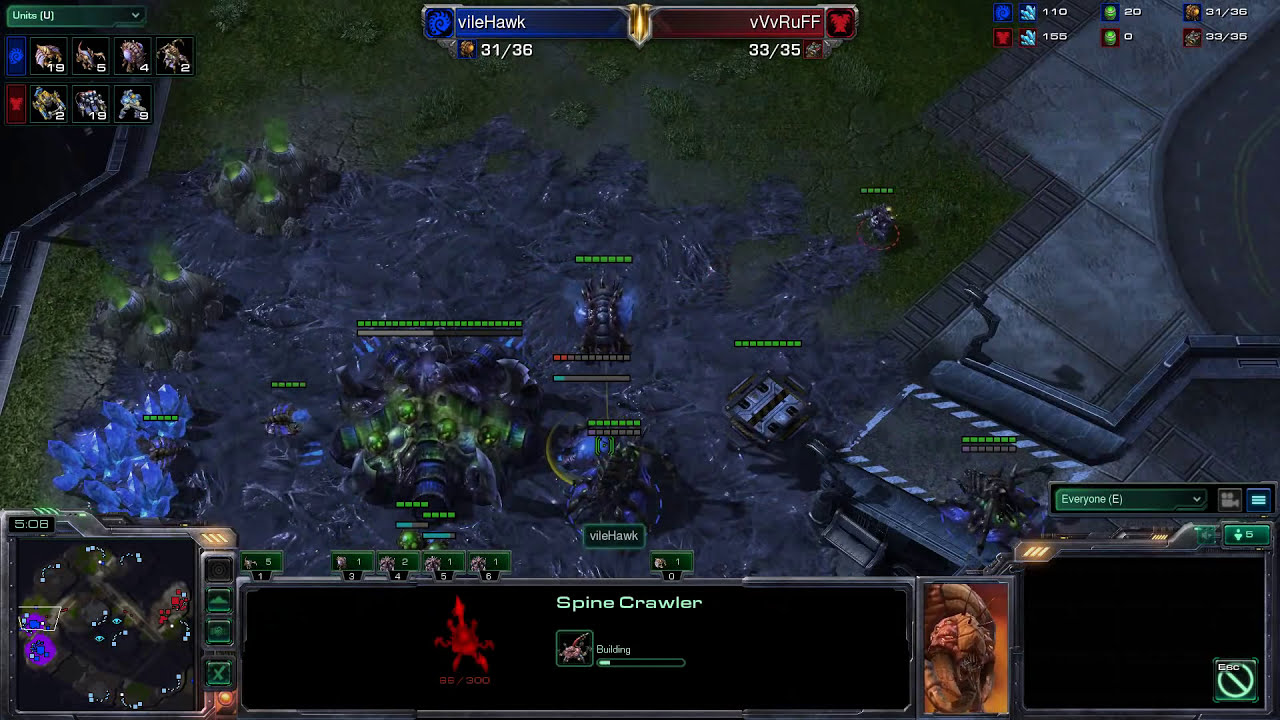This image is a screenshot from a real-time strategy (RTS) video game with a futuristic sci-fi theme. It features a top-down view of the battlefield where two teams, represented by players Vilehawk (blue team) and VVVRUFF (red team), are engaged in combat. The names of the players are displayed at the top of the screen against blue and red backgrounds, respectively, and the center features a gold icon.

The image depicts a gray central area with a field of green surrounding it, and to the right, there is a track-like structure. Several characters with green health bars above them can be seen battling, with the central character named "Spinecrawler." This name is highlighted in green text in a black box at the bottom center of the screen. 

In the bottom left corner, an overhead map displays the base camps of both the blue and red players along with various player positions, buttons, and the game timer. The interfaces include white text indicating player stats: Vilehawk "31/36" and VVVRUFF "33/35." The screen also features green and blue buttons along the edges and various game structures and vehicles with formations marked by green dots on top.